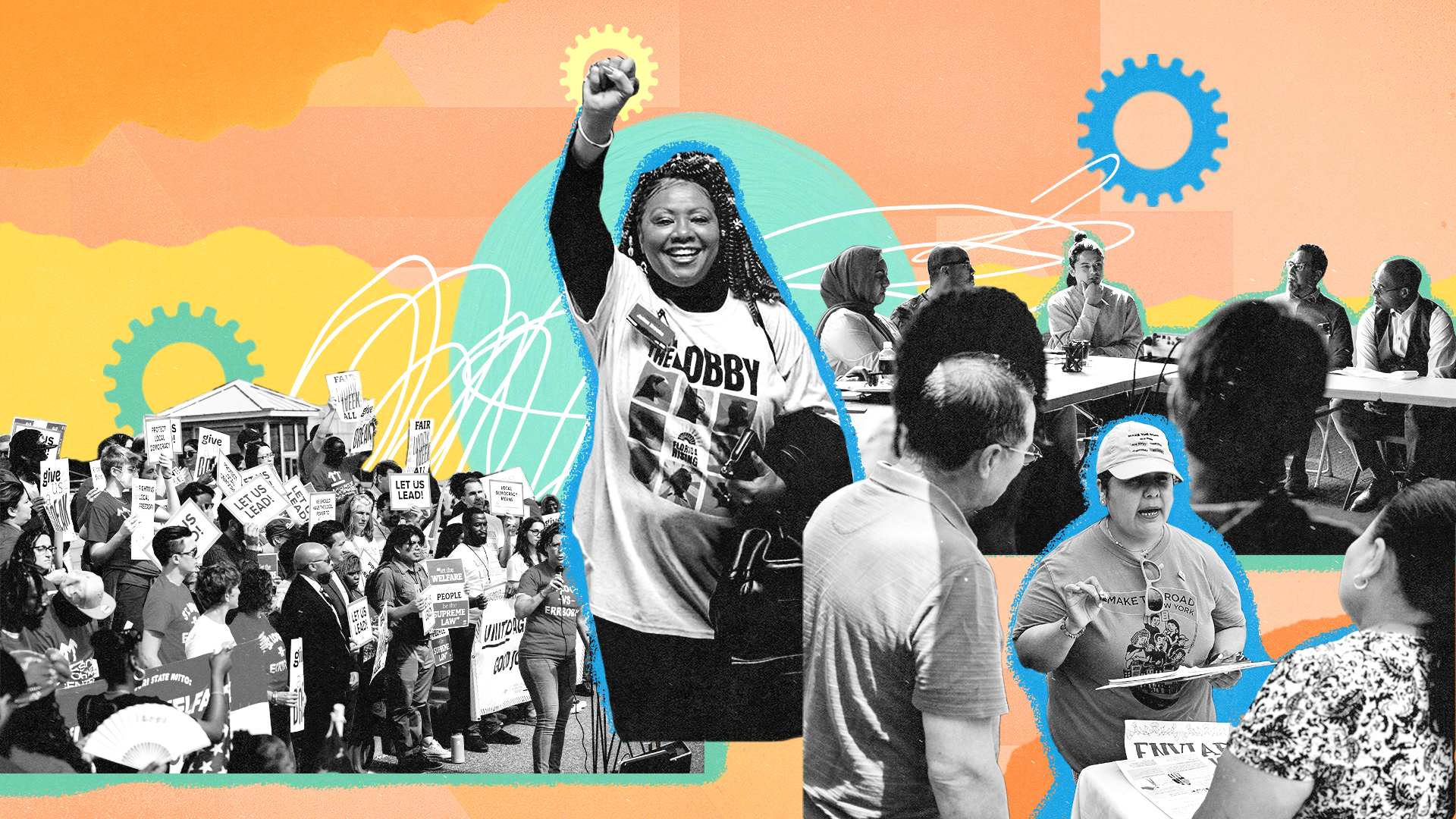The image features a detailed and vibrant panorama composed of various scenes related to justice, equality, and government, set against a backdrop of orange and peach tones, suggesting an illustration or graphic design project. Prominently in the center, a sepia-toned photograph depicts a historical women's suffrage march, with women donning capes and holding signs that read "We Demand Justice" and others that are partially obscured. Encircling this central protest image are elements symbolizing unity and contemporary collaboration.

At the top, numerous hands, rendered in black and white, clasp together in a display of solidarity. Below these hands, a prominent banner with an orange background and white lettering proclaims "Power and Potential." To the right of this central march, a black-and-white image of a government building adorned with a large American flag suggests a location in Washington, D.C. Below the building, a black and white scale, slightly tipped, symbolizes the quest for balance and equality.

On the left side of the image, two individuals with short hair, one with hair in a bun, are depicted in black and white, warmly embracing beneath a black bullhorn, representing activism and vocal advocacy. Nearby, three individuals, two seated at a desk and one standing, are engaged in collaborative work, their diverse backgrounds and attire reflecting modern inclusivity. The desk is cluttered with notebooks and a laptop, indicating a busy, interactive environment. Just to the right of these figures is a light brown rectangular object with a dark brown "3" and "717."

Overall, this rich composition intertwines historical and modern elements, showcasing a continuum of the fight for justice and equality amidst a blend of warm, inviting background hues.